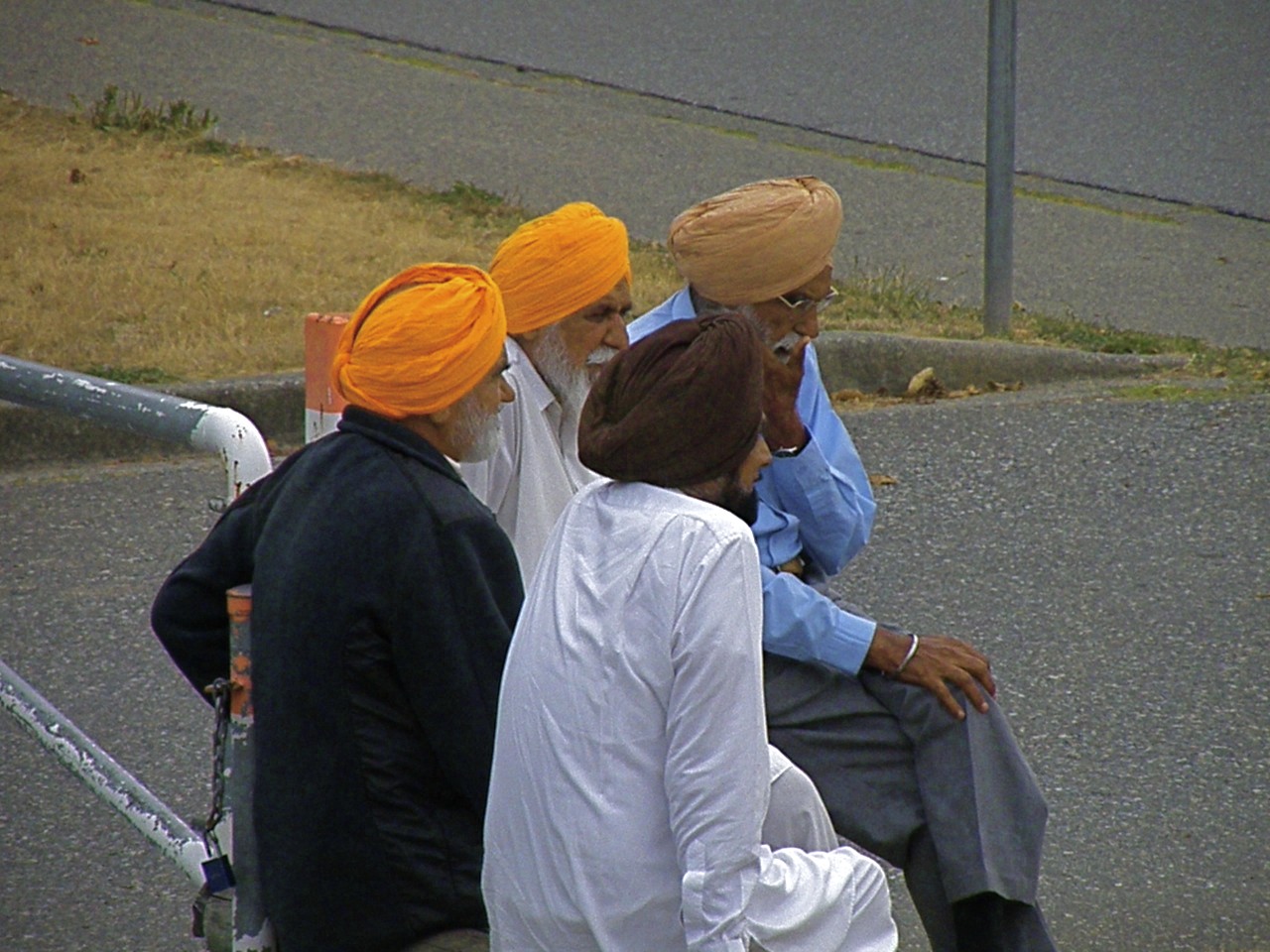The image captures an outdoor scene on the side of a road, depicting four elderly men, likely in their late 50s to 60s, seated close together on the concrete ground. Each man is adorned in a distinctive turban, suggestive of a Muslim background. Two of the turbans are a bright orange, one is a dark brown, and the fourth is a beige or peach color. 

The men are engaged in a conversation, with the one in the blue collared shirt appearing contemplative, his right hand resting on his face. He is noticeable with his glasses, silver bracelet, grey pants, and black socks, and has his legs crossed. One of the men in a bright orange turban is dressed in a black fleece jacket, while another in a similar turban wears a white shirt. The man in the dark brown turban is clothed in a long white robe.

The setting includes a dark grey road, a white and grey pole visible towards the top right, and some patches of faded grass, hinting at a roadside or the perimeter of a property. The atmosphere suggests a casual yet thoughtful gathering, possibly highlighting a moment of communal discussion or reflection.